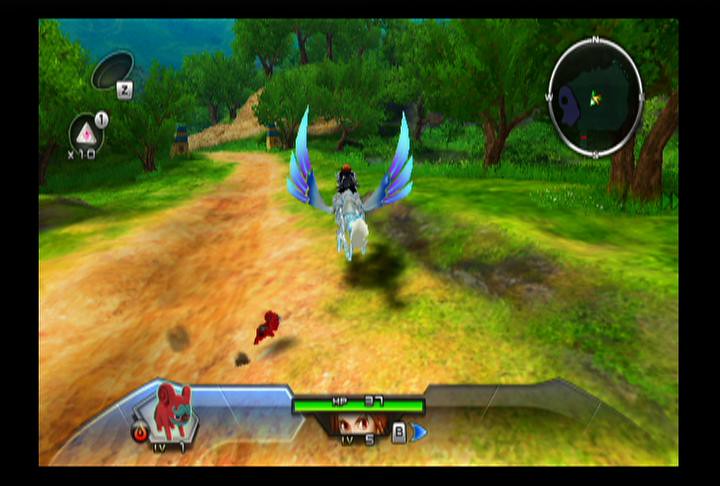The image is a screen capture from a video game, depicting an outdoor scene on a dirt road flanked by green grass and trees on both sides. In the center of the image, a character with brown hair dressed in a black suit is riding a creature that resembles a winged horse. The creature has purple-blue wings and a white tail, and it appears to be flying, casting a shadow on the ground. Below the character, there's a small, red, dog-like monster that seems to be chasing after them. The user interface (UI) overlays the bottom of the image, displaying the character's face, their level (5), and their hit points (HP 27). On the left side of the UI, there's an icon of the red creature labeled as level 1, accompanied by a small fire symbol. The top left corner of the screen features some icons and numbers: a 'Z' button, the number '1,' and a triangle with '×10' underneath it. The top right corner displays a mini-map. The overall graphics are somewhat blurry and primitive.